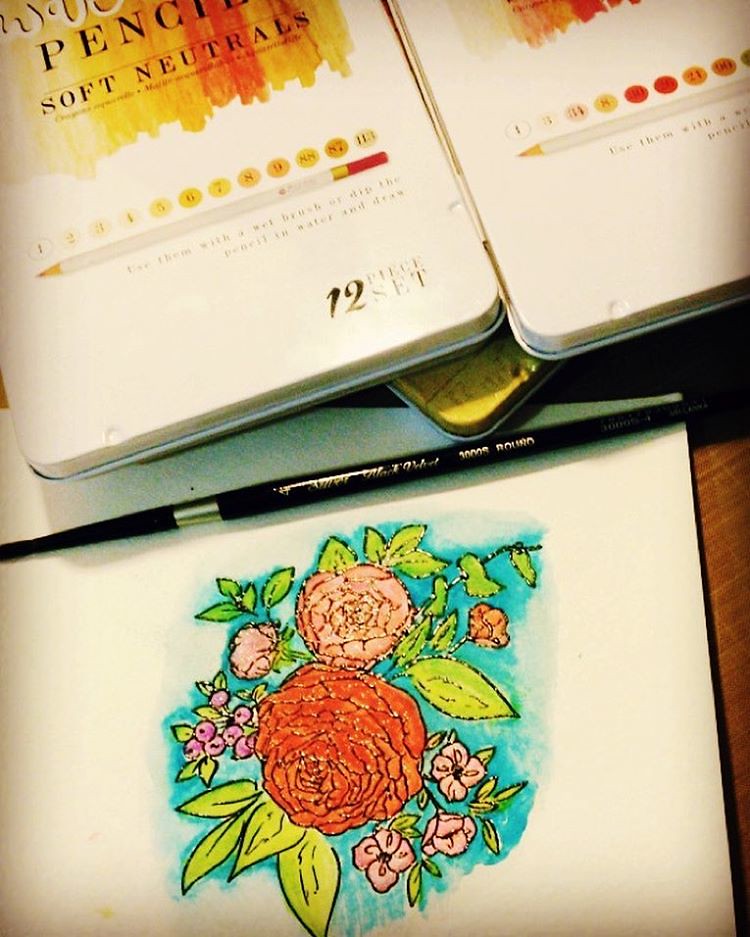This indoor, color portrait photograph depicts a detailed still life scene of drawing materials arranged on a darkish brown wooden table. Dominating the lower half of the image is a white sketchpad showcasing a pencil drawing of a small bouquet. The bouquet, rendered in precise detail, features a pink rose paired with a darker red rose near the center, surrounded by a mix of green leaves and purple berries, with smaller light pink flowers accenting the composition. The bouquet is set against a bare white background with a hint of light blue, perhaps representing the sky. A black pencil with silver writing lies diagonally across the page, accentuating the artistic theme.

In the upper half of the image, two identical tan-colored tins containing drawing pencils are displayed side by side. These tins, labeled with the words "soft naturals" and "12-piece set" in gold lettering, are partly opened to reveal the profile of the pencils inside. The entire scene is in sharp focus, emphasizing the intricacy and richness of the drawing materials and the artwork itself.